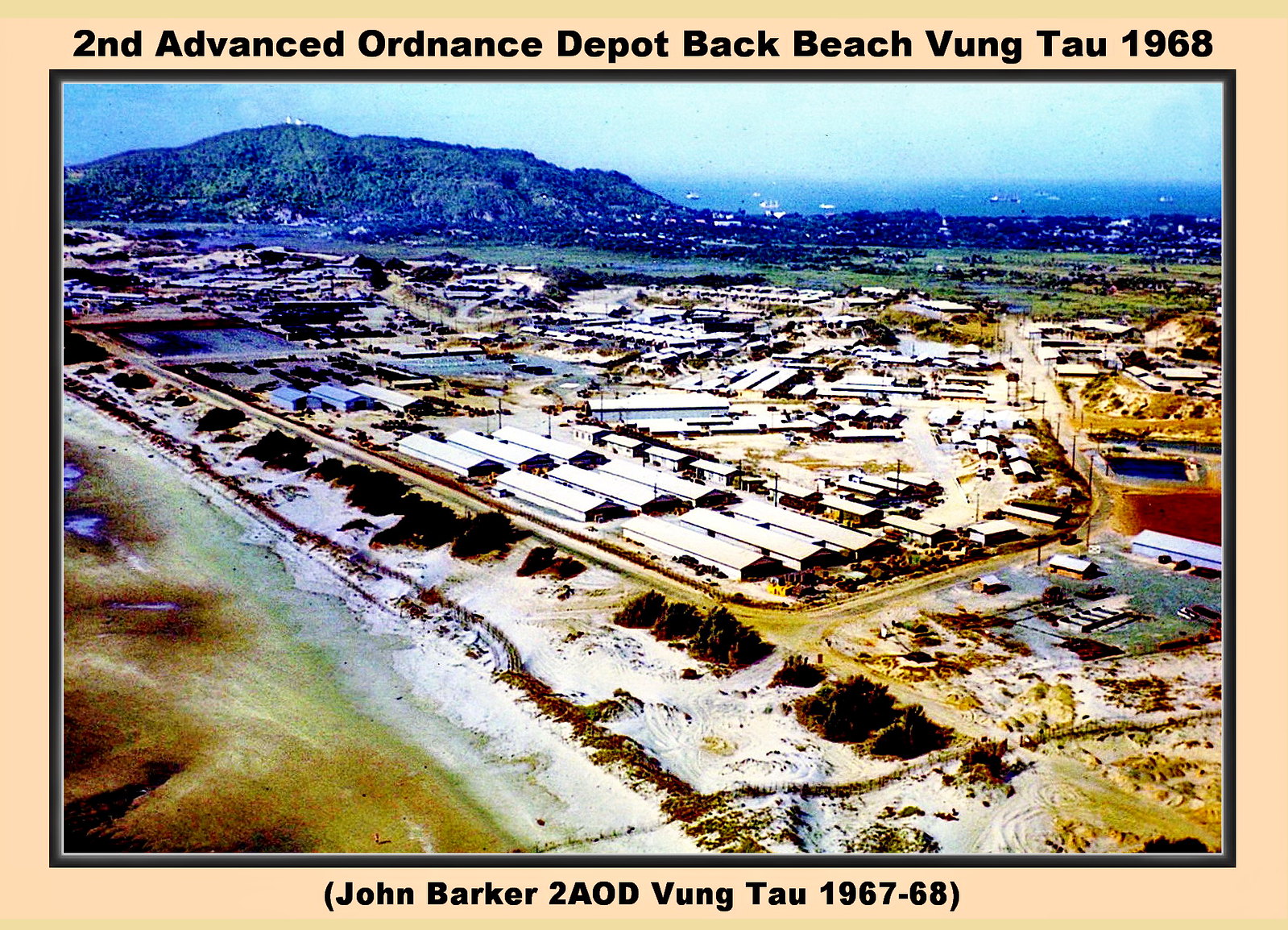This vintage 1968 photograph, marked as "2nd Advanced Ordnance Depot, Back Beach, Vung Tau" and credited to John Barker (2AOD, Vung Tau, 1967-68), offers a high-angle aerial view—likely taken from a helicopter during the Vietnam War—of a developed, industrial area adjacent to a long, sandy beach. The beach is deserted, demarcated by a fence line stretching across its length, suggesting restricted access, possibly for military purposes. Numerous long, steel warehouse-like buildings are clustered together, with several roads and visible electric and telephone infrastructure weaving through the area. The surrounding landscape includes a small, tree-covered mountain and additional ocean waters in the background, pointing to the location being an island-like area. The photograph, now faded and tinged with brown hues, is bordered in deep gray and cream, enhancing its historical and worn aesthetic.